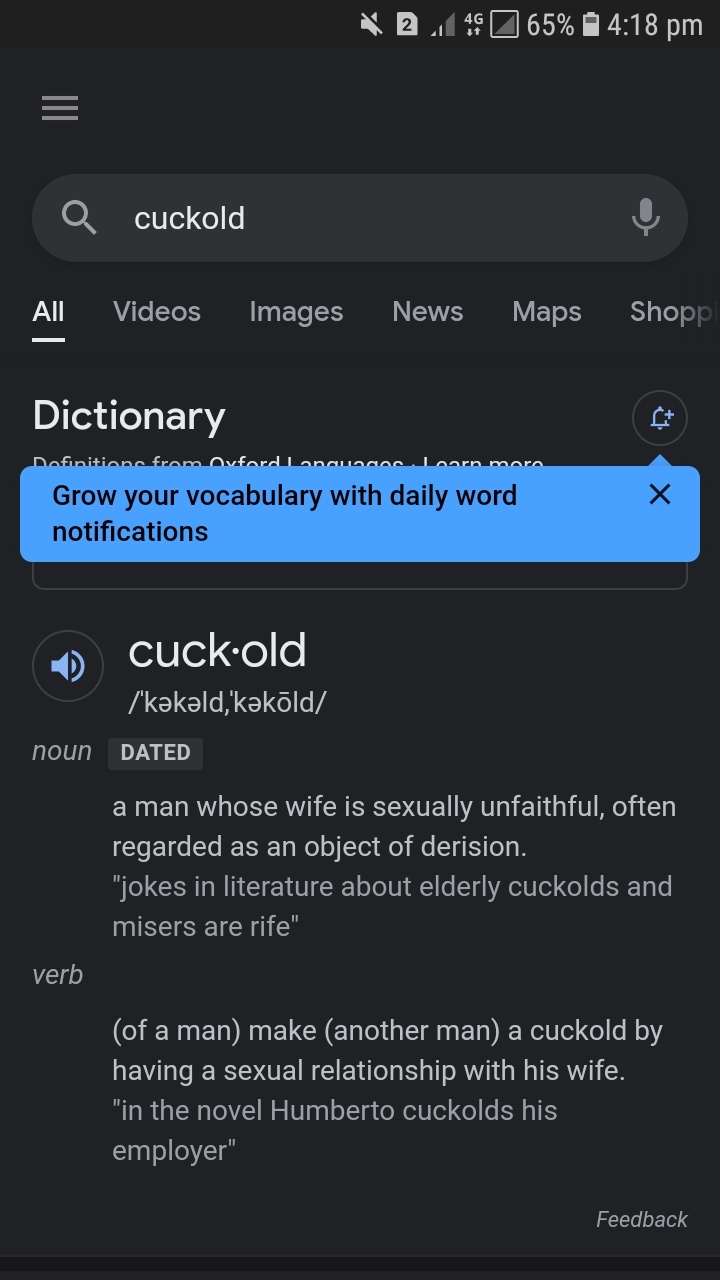This screenshot captures a dictionary entry viewed on a smartphone. The background is black, providing high contrast for the white text. At the top, the search area contains the word "cuckold" in white. Below the search bar, navigation categories are displayed horizontally, including "All," "Videos," "Images," "News," "Maps," and "Shop," with the "All" category highlighted, underlined in white text. 

Directly beneath, the word "dictionary" is prominently displayed in white text. Following this, there is a notification prompt in a horizontal rectangular area, reading "Grow your vocabulary with daily word notifications" in black text, accompanied by a black 'X' in the upper right corner to dismiss the prompt. 

The main content begins with the word "cuckold" in bold white text, followed by its phonetic pronunciation, also in white. The term "dated" is indicated in white text, while "noun" is displayed in gray text along the left margin. The definition provided reads: "a man whose wife is sexually unfaithful, often regarded as an object of derision. Jokes in literature about elderly cuckolds and misers are rife." 

Additionally, the entry includes a verb form, also in gray text along the left margin. The definition for the verb form states: "of a man, make another man a cuckold by having a sexual relationship with his wife. In the novel, Umberto cuckolds his employer." 

At the bottom right of the screen, a small button is labeled "Feedback" in white text.